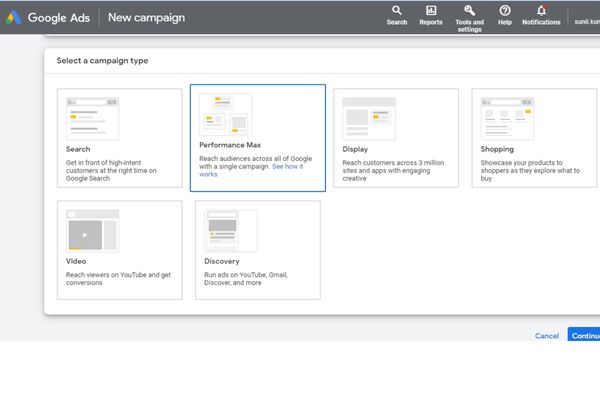Screenshot Description:

In the screenshot, the visual layout begins from the top left corner to the upper right, featuring a primarily dark gray background. The top area is adorned with a series of navigation elements from left to right: starting with a green V-shape that transitions into yellow and eventually blue. Adjacent to this colorful sequence, there are white text labels reading "Google Ads new campaign." Moving rightward, other navigation options include "Search," "Reports," "Tools and Settings," "Help," and "Notifications."

Beneath the dark gray backdrop, there's a prominent white box with black text that reads "Select a campaign type." Below this, there are four horizontally aligned boxes:

1. **Search** - Encased in a gray outline, this option emphasizes "Get in front of high-tech customers at the right time on Google Search."
2. **Max Performance** - Outlined in black, this option details "Reach audiences across Google with a single campaign. See how it works."
3. **Display** - Surrounded by a gray border, it invites users to reach "customers across three million sites with apps and engaging creative."
4. **Shopping** - Also surrounded in gray, this option aims to "Showcase your products to shoppers as they explore what to buy."

Below these, there are two additional horizontally aligned options on the next row:

5. **Video** - Emphasized to "Reach viewers on YouTube and get conversations."
6. **Discovery** - Allowing users to "Run ads on YouTube, Gmail, Discover, and more."

At the bottom right of the screen, there are two clickable buttons: a blue "Cancel" button and a prominent white "Continue" button edged in blue.